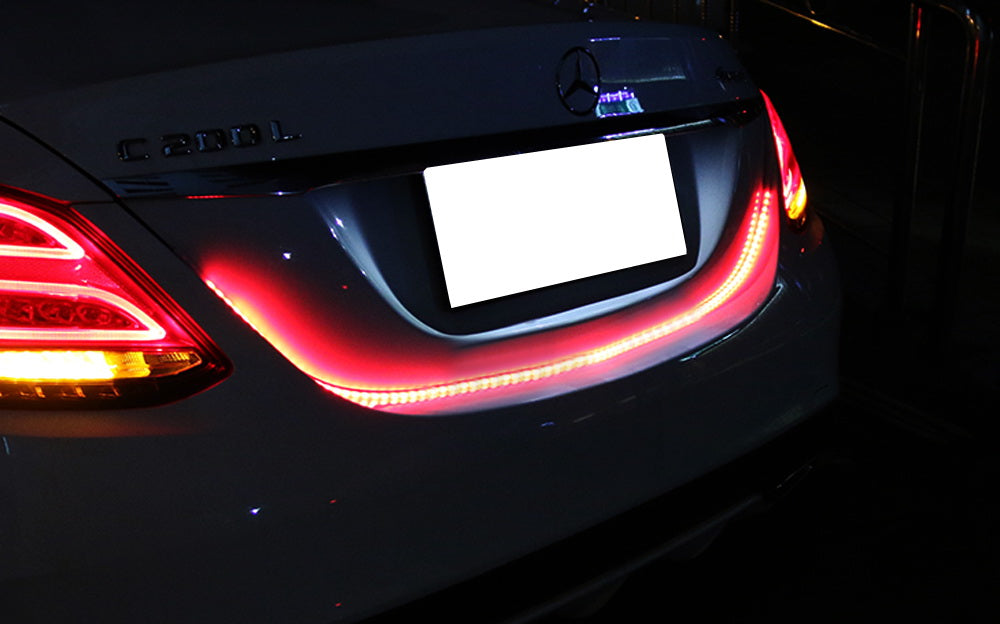The image showcases the rear of a Mercedes-Benz C200L, photographed at night. The specific model designation, "C200L," is clearly visible on the left side of the trunk lid. A prominent Mercedes emblem is centrally located on the trunk. The taillights are illuminated with a primarily red hue complemented by an amber color at the bottom. Additionally, the area where the trunk meets the car body is highlighted with distinct LED lights, suggesting a custom design element. The license plate area is glowing with a white light, but the actual license plate is not visible. The scene is dark, with the only other discernible details being tiny light reflections on what seems to be a wall in the background, located in the top right corner of the image. The car's exterior color is indiscernible due to the darkness surrounding the vehicle.